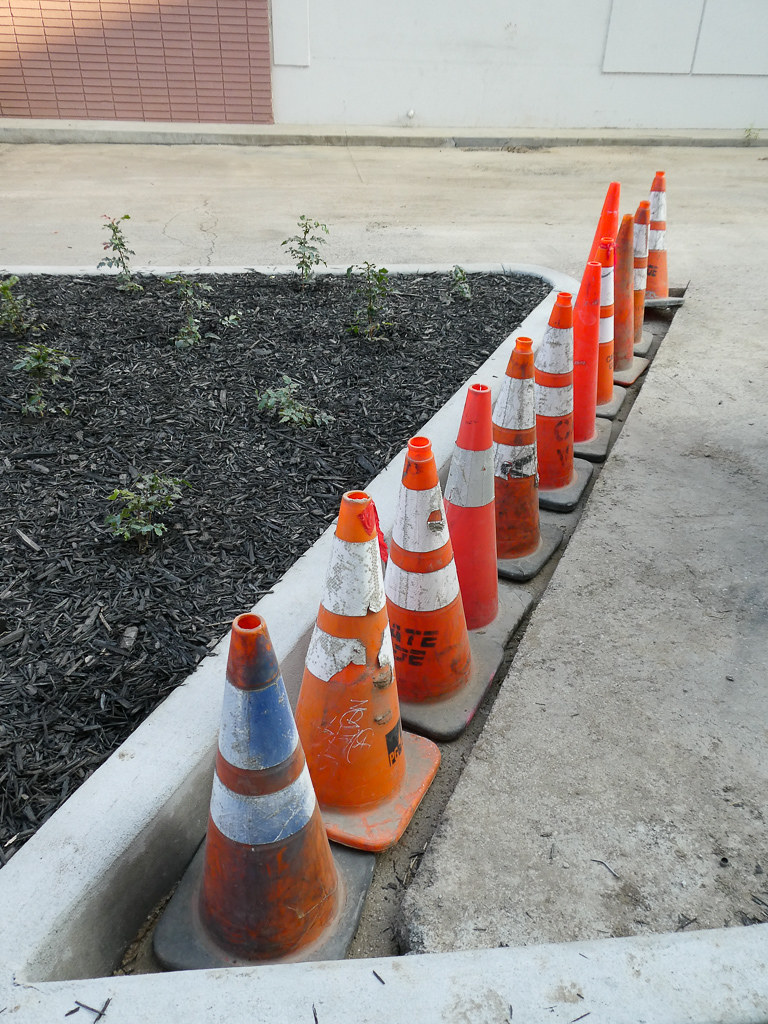This image depicts a row of approximately 11 orange traffic cones, each with two white stripes near the top and a grey-colored flat base. These cones are positioned along the edge of a lowered cement area that resembles a drain or trough, below the main ground level. Behind the cones is a raised partition filled with black mulch and newly growing green plants. The background showcases a dichotomy in the surroundings: to the left, there is a reddish brick wall, while to the right, a plain white wall is visible. Further back, a dark greyish sidewalk or road curves upward and around, defining the boundary of this planted area amidst urban infrastructure. Some cones appear scratched or marked, with variations in their orange hues.